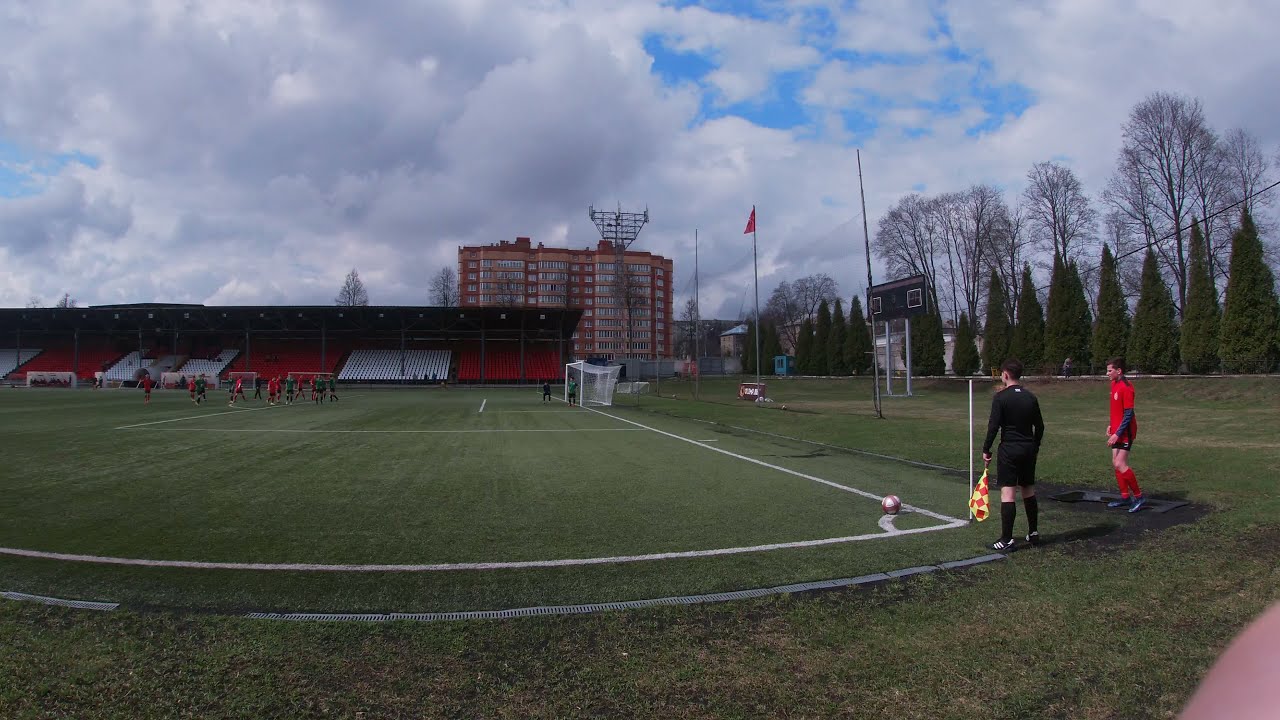This detailed photograph captures a vibrant scene on a professional or college-level soccer field, covered with lush green grass and marked with crisp white lines defining the boundaries and boxes. Dominating the right-hand side of the image, a player in a red and blue uniform is poised to kick a soccer ball positioned in the corner. Nearby, an umpire dressed in black, holding a flag, stands attentively. Further in the background, several other players are visible across the expansive field. The stadium itself boasts red and white bleachers filled with spectators, indicative of a lively match. Adjacent to the stadium is a multi-story building painted in red and cream hues. The scene is set under a mostly cloudy sky with patches of blue peeking through, while the boundary of the stadium is lined with neatly planted trees, adding to the serene ambiance of the setting.